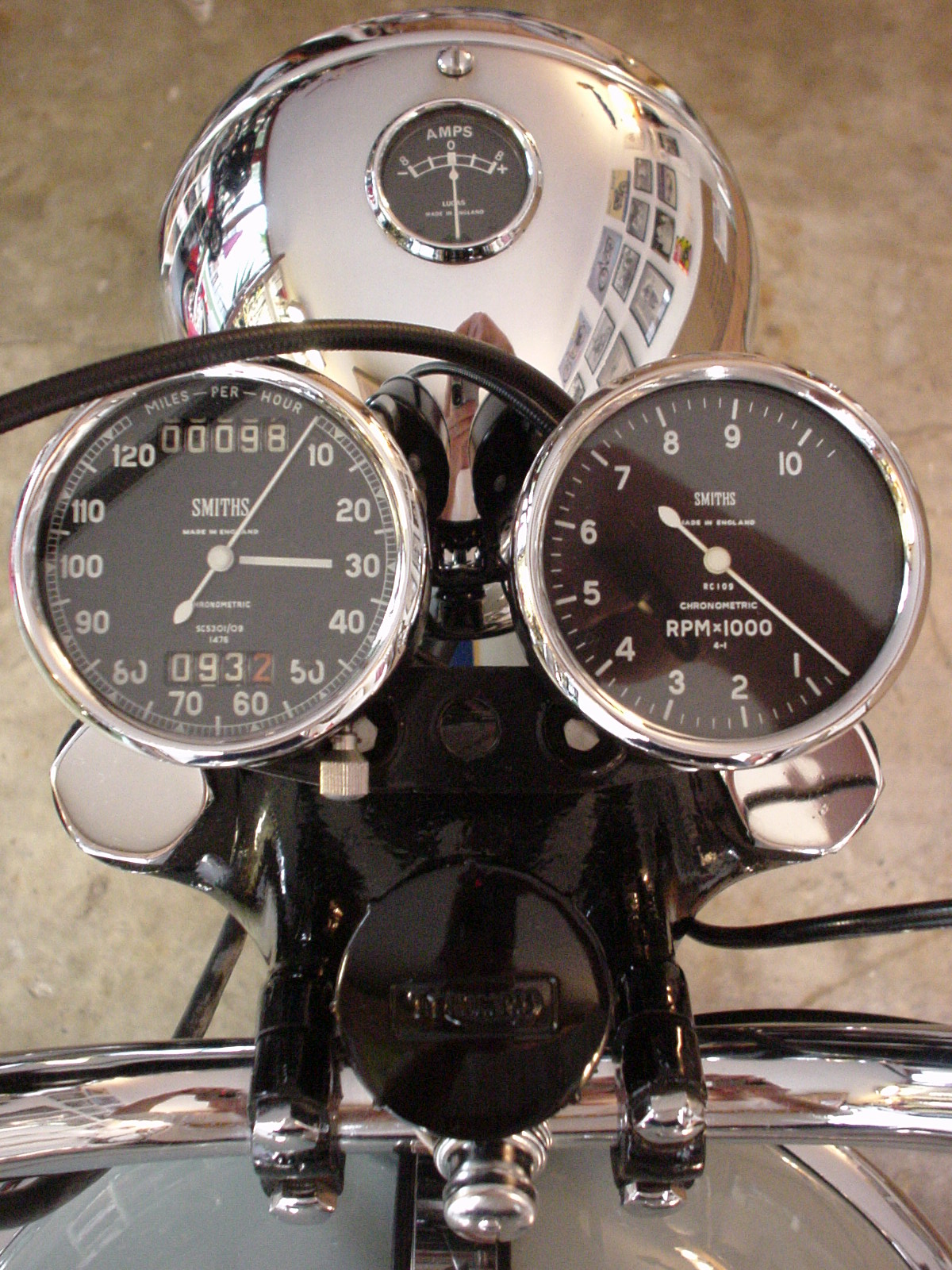The image depicts a detailed view from the rider's seat of a motorcycle, focusing on its front end. The motorcycle is stationed on a light brown concrete surface, possibly a driveway or the inside of a garage. Central to the image is the gleaming silver front of the motorcycle, which is exceptionally shiny. Featured prominently at the top is a slightly duller, triangular silver section. 

The focal point includes a large silver circle housing an ammeter, characterized by white letters spelling "AMPS" on a black background, with a needle to register the amperage. Adjacent to this, a thick black hose is visible. Next, there's another prominent silver circle containing a speedometer, with its inner section in black, and yet another large silver circle showcasing an RPM gauge, also black inside with white numbers. Below these instruments, the gas cap is noticeable, distinctively black. Also visible are the supports for the windshield, rising from the bike's body, completing this intricate portrayal of the motorcycle’s dashboard area.